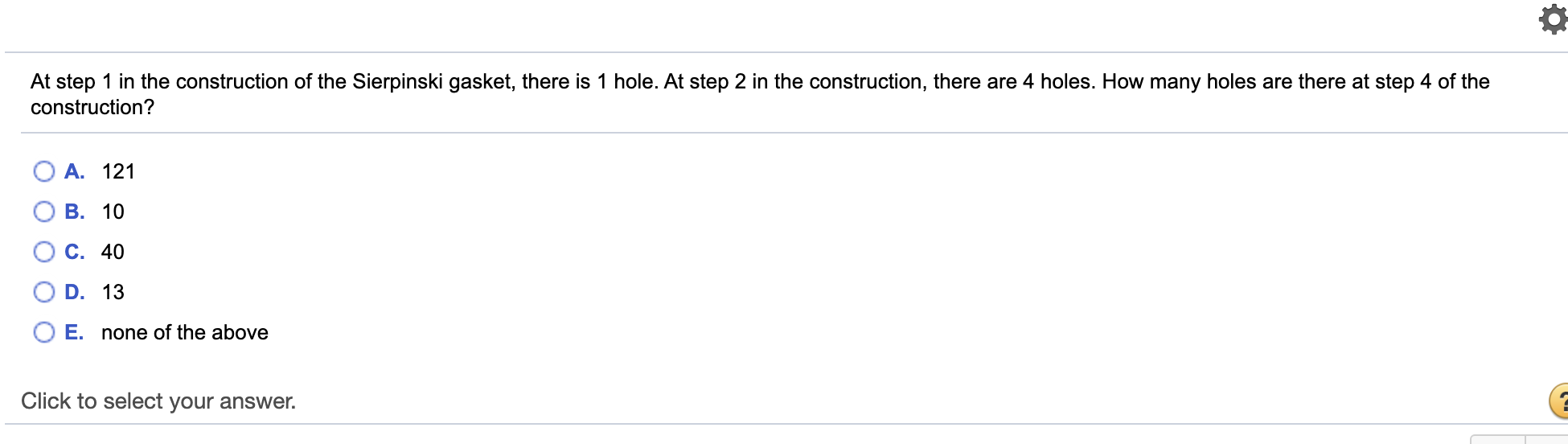This image captures a webpage viewed on a digital device, displaying a problem related to the construction of the Sierpinski gasket. At the top, a thin gray line spans the width of the page, with a dark gray gear icon situated at the far right. Below this line, text appears in black, detailing the construction steps of the Sierpinski gasket:

- "At step 1 in the construction of the Sierpinski gasket, there is 1 hole (1)."
- "At step 2, there are 4 holes (4)."
- A question follows: "How many holes are there at step 4 of the construction?"

Beneath the question, possible answers are listed as bulleted points, each prefaced by a blue circle containing a letter:

- A. 121 (in black)
- B. 10
- C. 40
- D. 13
- E. None of the above

Immediately below these options, a prompt in black text reads, "Click to select your answer."

A gray line separates this section from the rest of the webpage. To the right side, an orange circle features a blue question mark inside it. Below this, partially cut off, is a small gray area that appears to be a button.